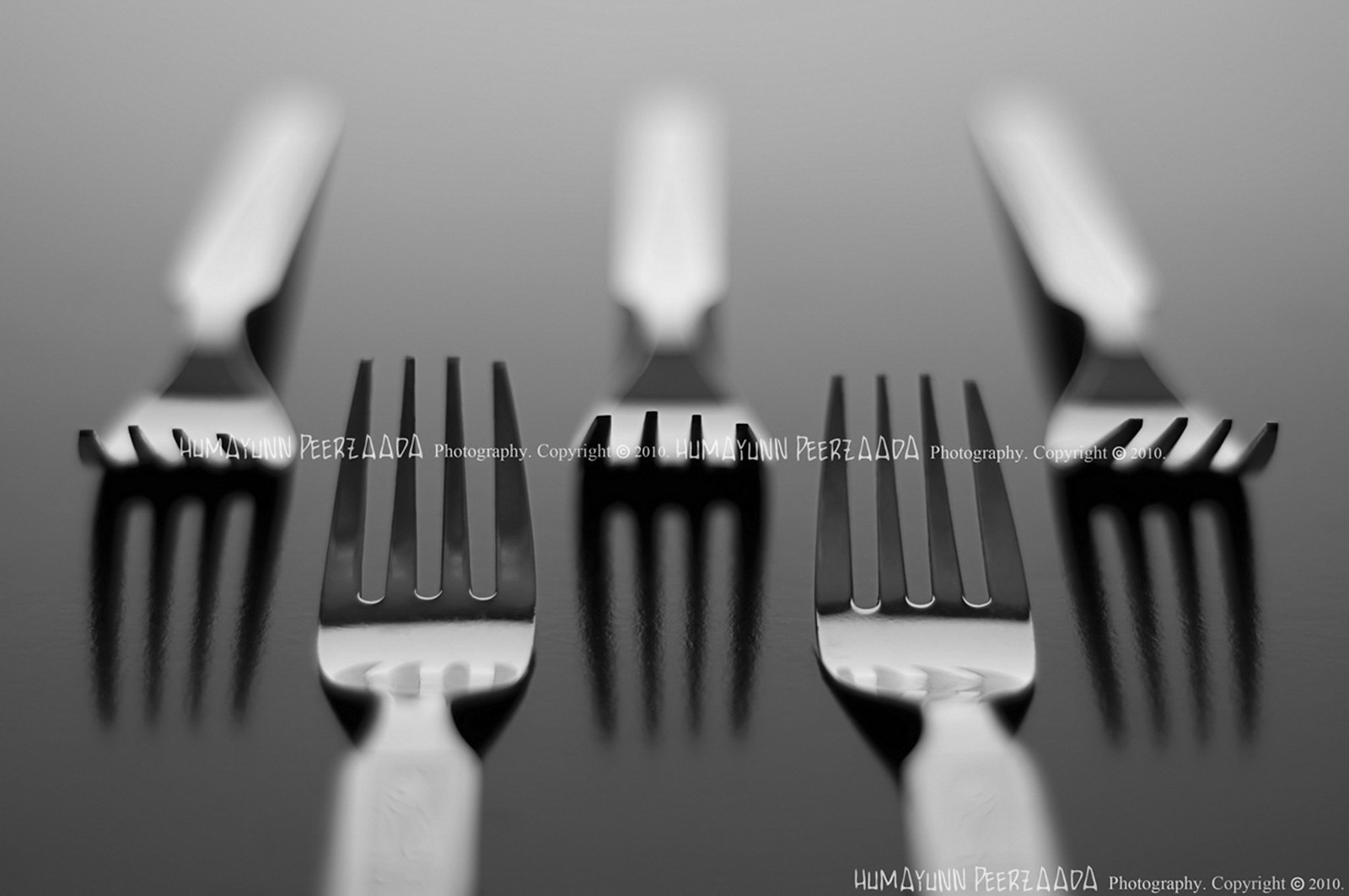The image is an artistic black and white photograph featuring five silver forks, arranged with alternating handle directions. The main focal point of the photograph is the tines of the forks, three of which are facing towards the viewer, while two extend away from the bottom. The photograph exhibits a shallow depth of field, rendering the top portions of the forks extremely blurred. The handles, whether oriented towards the top or bottom, fade into a gray background with significant blur. Shadows are cast by some forks, adding a dynamic element to the composition. There are white watermarks across the center and bottom right of the image, indicating the photographer's name: Humayun Peerzada, with a copyright mark for the year 2010.